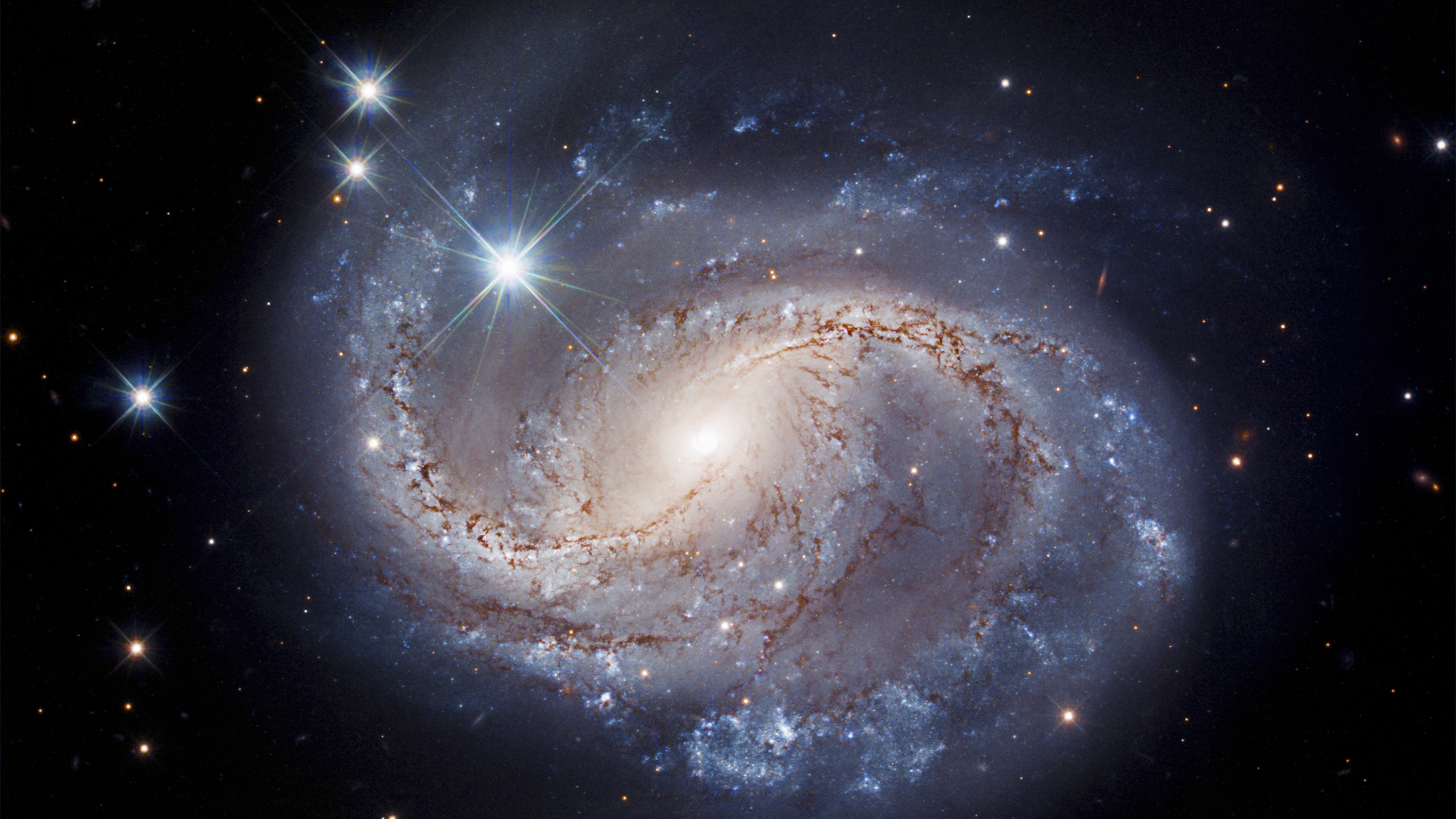This image captures the breathtaking beauty of deep space, featuring a prominent swirling galaxy with a mixture of white, blue, and brown hues. The galaxy's form is intricately composed of numerous tiny stars, enveloped by dust clouds from various nebulas. At the heart of the galaxy is a dazzling, bright center, radiating light that spirals outward. Scattered across the top right and top left of the image are four exceptionally bright stars, each emitting striking light rays in multiple directions. The backdrop is a vast black sky peppered with stars of various colors, including red, orange, white, and off-white, emphasizing the contrast between the larger, shining stars and their smaller, fainter counterparts. This photograph masterfully captures a whirlpool-like galaxy, reminiscent of the Milky Way, revealing the grandeur and complexity of the cosmos.